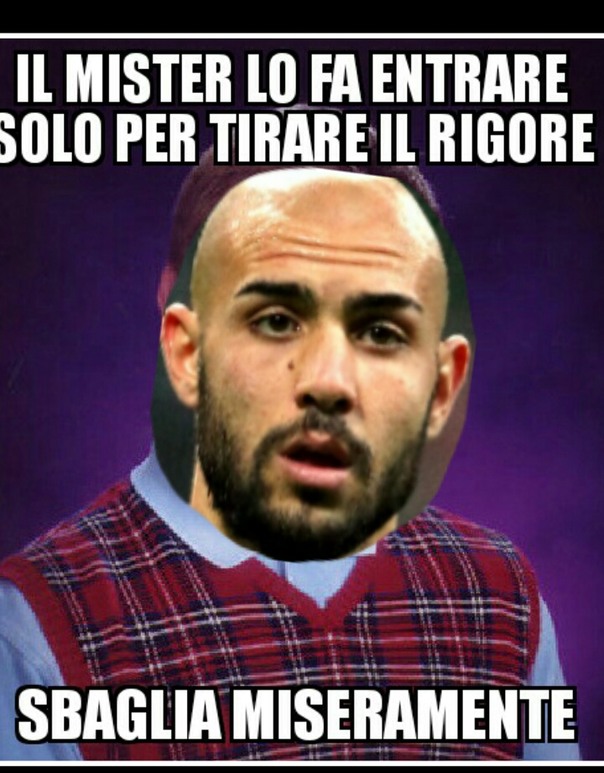The image features a person dressed in a blue collared shirt and a red plaid vest, the plaid incorporating blue, white, and red colors. Over the original face, another face has been superimposed—a bald man likely in his late 30s, characterized by dark eyebrows, a beard and mustache, and a distinct mole beside his nose. He has an expression that could be described as slightly baffled. The backdrop appears to be a typical school photo setting with a purple background. Across the top of the image, there is text in a foreign language that reads, "El Mister Lofa Intrare Solo Per Terare El Rigor," and at the bottom, "Sabaglia Misurmente." This alteration seems to stem from a humorous meme, juxtaposing the incongruous face onto the original photo subject.